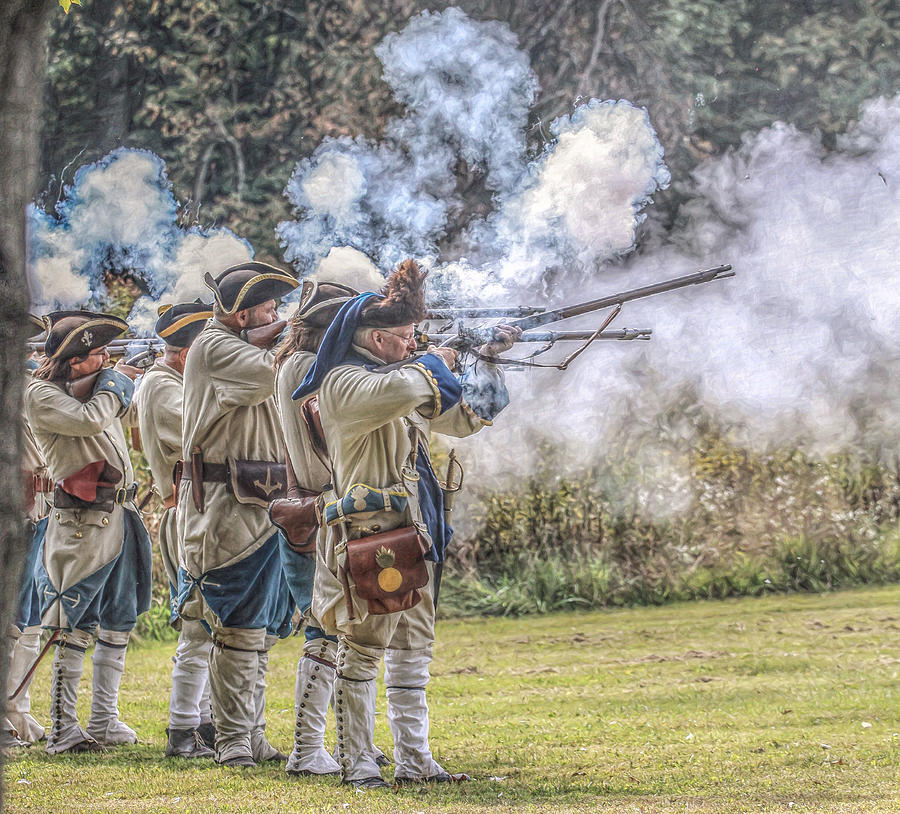This image captures a detailed scene from a Revolutionary War reenactment. Five men, all in Colonial-era uniforms, form a line as they fire their long muskets simultaneously, generating thick white smoke that hangs in the air. Each man sports a black tricorn hat with a gold or white trim. Their attire includes tan long-sleeved jackets with blue and gold cuffs, complemented by tan pants featuring a blue stripe and white knee-high socks under tan boots adorned with buttons down the sides. Accessories include leather belts holding pouches and possibly knives. The background is a lush landscape filled with a variety of green elements, including brush, taller grasses, and several trees, one notable large limb extending on the left side. The scene is set in a mowed grassy field, and there are no text or numbers visible, focusing wholly on the historical tableau.